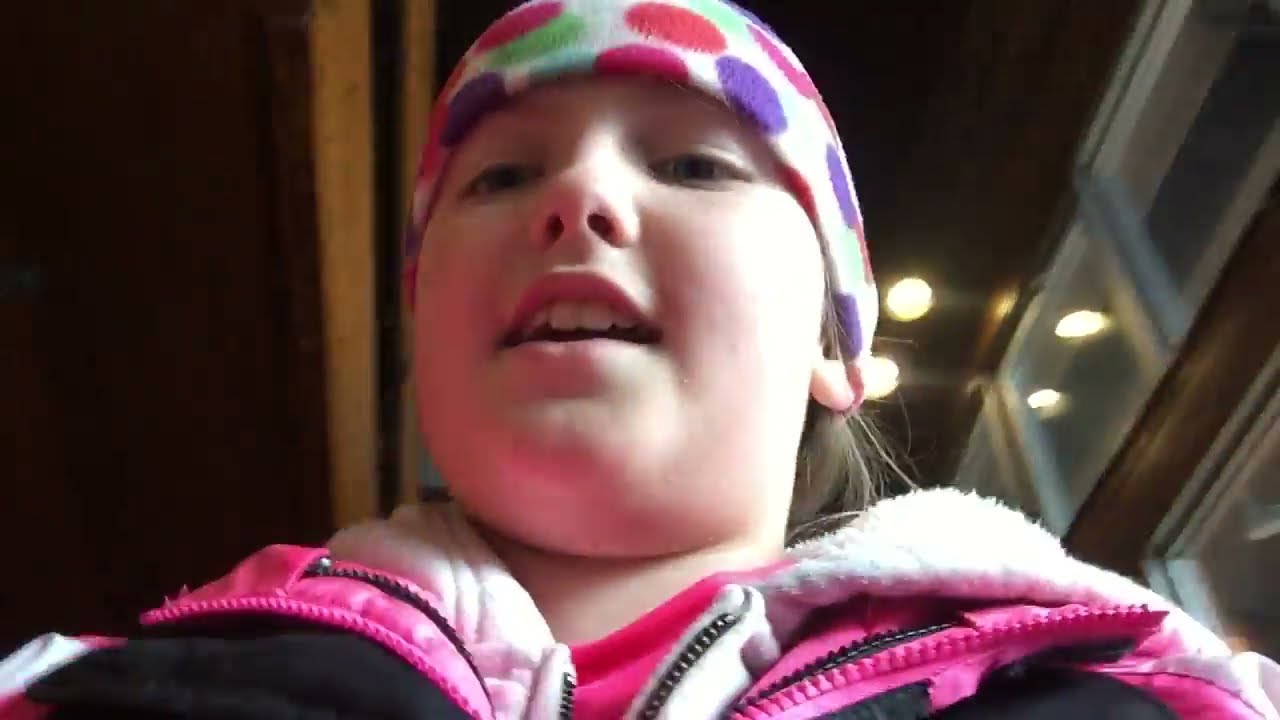The image portrays a young child, possibly a girl, who has taken a selfie. Her chubby, light-skinned face is prominently featured as she faces the camera, her mouth slightly open, revealing her top row of teeth. Her eyes are dark, with hints of lighter tones due to the lighting. She is wearing a warm, multi-layered coat composed of white, pink, and black, over a pink hoodie with a gold zipper. Atop her head is a white winter cap adorned with large polka dots in colors such as purple, red, hot pink, lime green, and turquoise. A few strands of her brownish-blonde hair peek out from under the cap. The photo is taken indoors, possibly in a room with a brown ceiling decorated with circular, fluorescent lights and wooden elements visible in the dim surroundings.